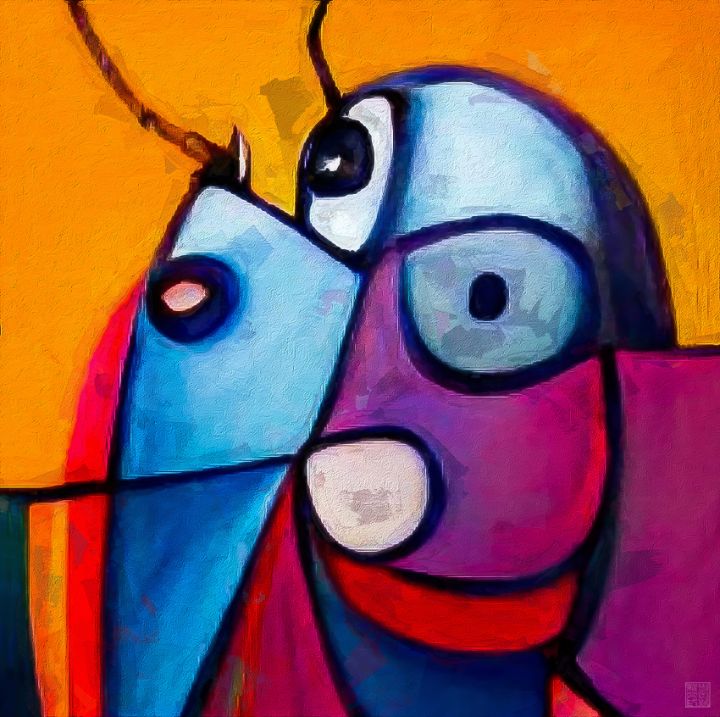This contemporary, modern art painting, reminiscent of Picasso's style, features an almost solid, textured dark yellow-orange background. At the forefront, abstract shapes are outlined with thick black lines and filled with an array of vibrant colors, including shades of blue, red, pink, and purple. The central figure appears disjointed and childlike, suggesting a creature that might resemble a dog or a bug. Its head, primarily white, has uneven round eyes—one pink and the other dark blue—with a white circle in the middle. A black, exaggerated nose or mouth seems shifted to the left, with a red stripe and blue shield extending downwards. The body exhibits more abstract forms, with a leg sticking out and various bright colors dispersed throughout, creating a visually engaging and textured piece full of unique shapes and intricate details.